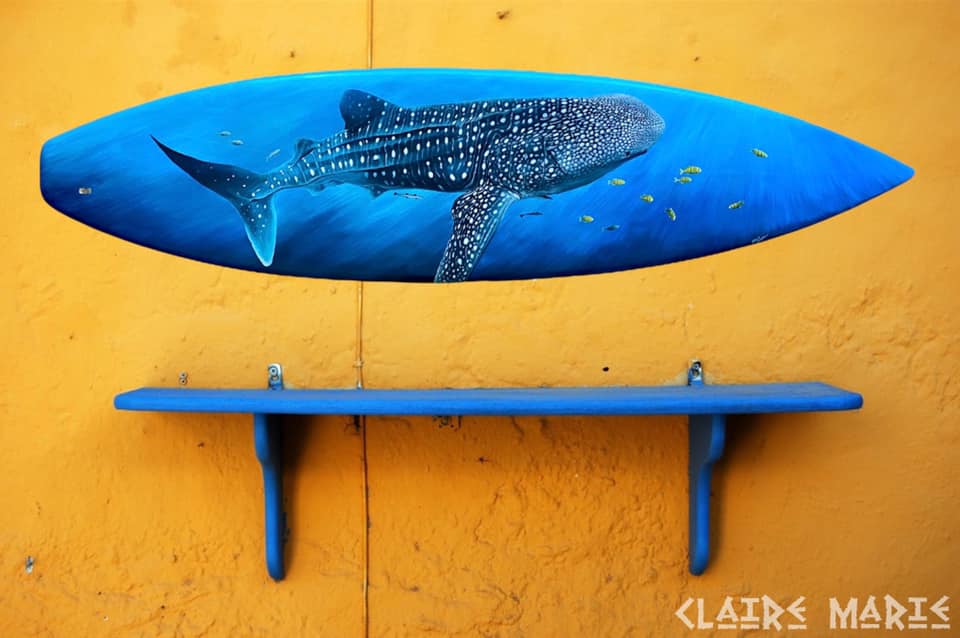The image depicts an indoor scene featuring a yellow painted, stucco-like stone wall adorned with a narrow blue bench and a similarly colored surfboard affixed above it. The bench, supported by two posts attached to the wall, appears rather thin, suggesting it might be uncomfortable to sit on. Above the bench, the surfboard takes center stage, painted in a vibrant blue reminiscent of neon sea hues. The surfboard's design showcases a prominent marine creature resembling a whale shark, dark gray with numerous spots, accompanied by smaller green and yellow fish. The background of the surfboard is painted to mimic water, complete with light blue streaks suggestive of sunbeams penetrating the surface. In the bottom right corner of the surfboard, white semi-transparent text reads "Claire Marie."